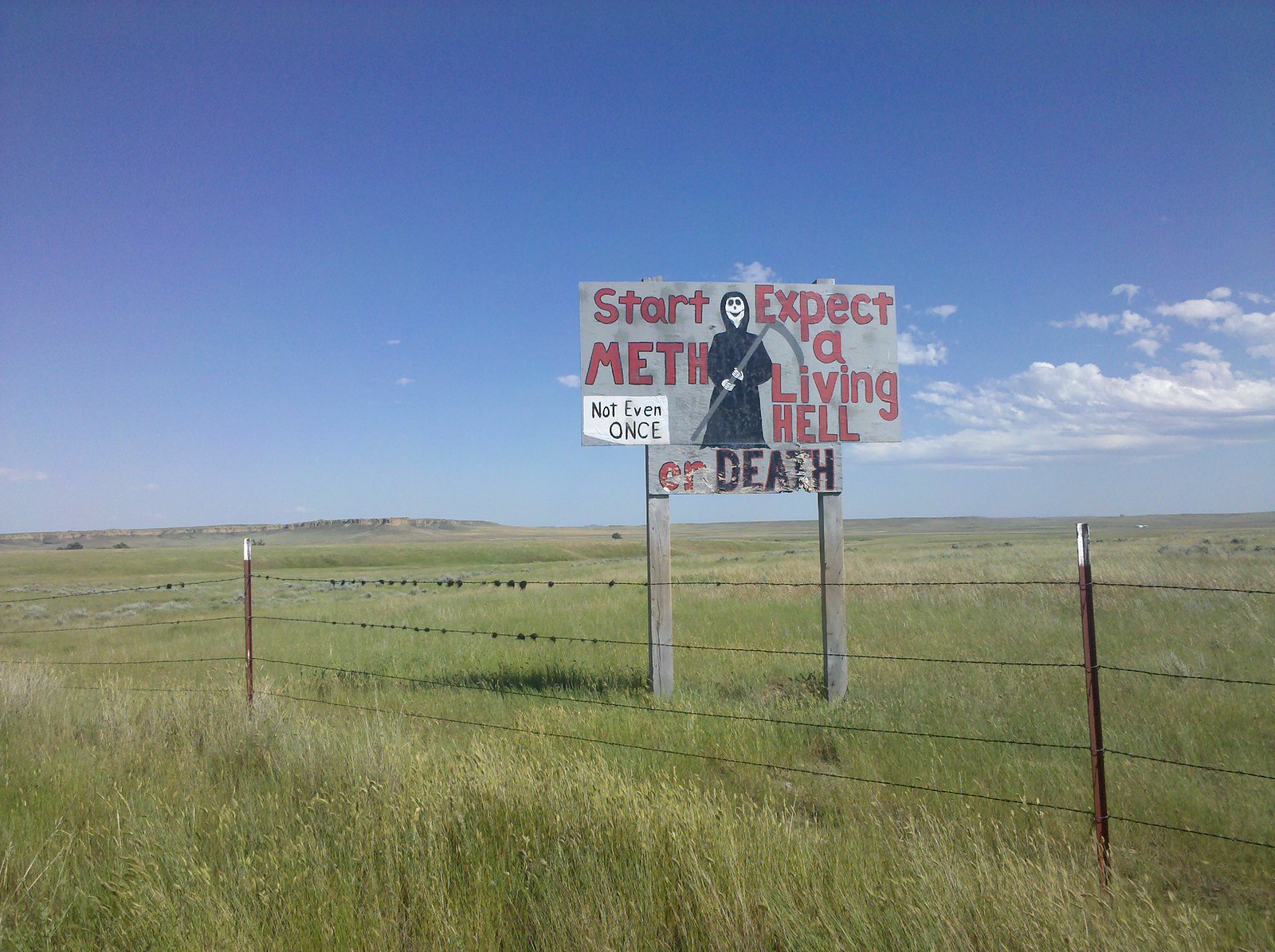In the image, there is a field enclosed by a weathered, wire fence that's certainly not meant to be trespassed. Behind this barrier stands a haunting, hand-painted billboard. The prominent message on the billboard is divided into three parts: "Start Meth" on the left, "Expect a Living Hell" in the center, and "or Death" at the bottom right—with the last part appearing scratched out and the wood chipped, giving it a particularly eerie feel. Adjacent to "Start Meth," a stark white box contains the bold, black text "Not Even Once," serving as a grim warning. Dominating the middle section of the board is a menacing Grim Reaper illustration. The Reaper, garbed in a flowing black robe and wielding a sharp scythe, grins ominously with his skeletal face, reinforcing the sinister message. The whole presentation of the billboard, with bubble-style red text and striking imagery, vividly conveys the dire consequences associated with drug use.